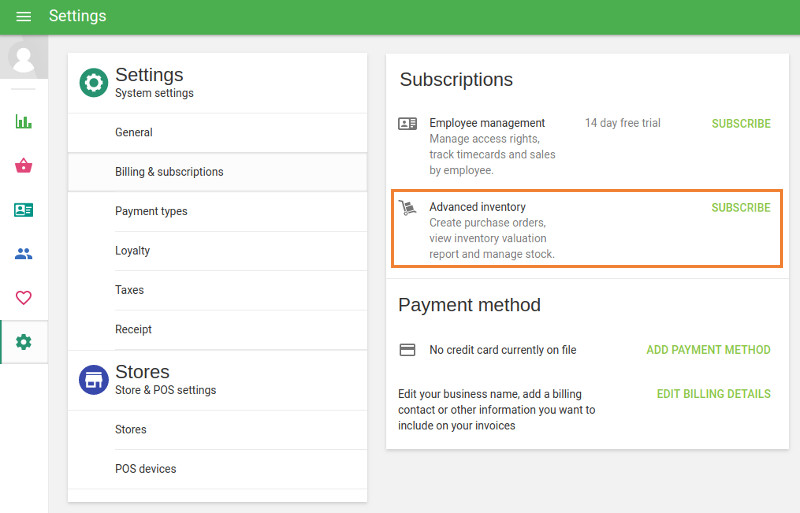At the top of the website's section is a bright green border. On the far left within this green section, there are three white horizontal lines, commonly indicative of a menu. Next to these lines, the word "Settings" is prominently displayed in white with a capital "S". Below this green section, there is a vertical white strip featuring a series of icons. These include a gray and light gray square with a white outline of a person, followed by a gray line. Below these, there is a green bar graph icon, a blue shopping bag icon, an icon resembling a tail ID, a blue outline of two people, and a dark pink heart icon. At the bottom, there is a highlighted section with a green gear icon, underlined by a green vertical line, set on a light gray background.

The user is currently in the Settings tab. The majority of the background is light gray, with two prominent rectangles. The first rectangle on the upper left includes a green circle with a white gear icon. Below this, in bold black text, it says "Settings" with "System Settings" underneath. A thin gray line separates the headings from more options below: General, Billing and Subscriptions, Payment Types, Loyalty, Taxes, and Receipts. The "Billing and Subscriptions" option is selected. Further below, the rectangle lists "Stores" and "Store and POS Settings." 

The second rectangle on the right starts with a header that reads "Subscriptions." Below this, it mentions an "Employee Management 14-Day Trial." The currently highlighted section is "Advanced Inventory" bordered by a garbage box. Further down, it states "Payment Method" with a note indicating "No credit card currently on file."